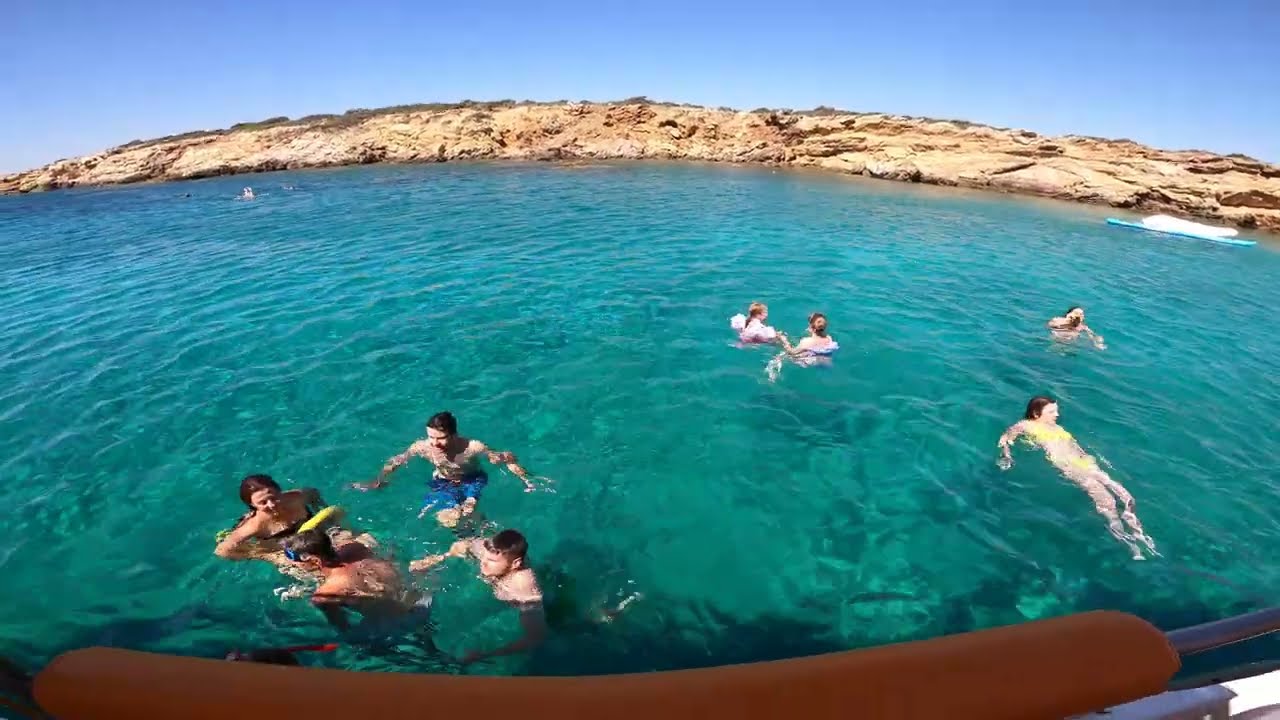This image depicts eight individuals enjoying the crystal-clear, light blue waters of what appears to be an ocean inlet or a large lake. The water is so transparent that the clarity creates a beautiful contrast with the surrounding environment. In the background, there's a rugged rock or dirt cliff formation marking the edge of the water, adding a dramatic natural backdrop to the scene. 

In the foreground, four people are huddled together in a circle, conversing or simply relishing each other's company. This group seems to be composed of one woman and three men. To the left of this cluster, there is a boat partially visible, suggesting that the group has ventured out from it and is now swimming leisurely in mid-water. 

Towards the center of the image, two women are seen floating in the serene water, embodying a sense of relaxation. Nearby, to their right, a man floats individually, slightly distanced from the others. In the bottom right-hand corner, a woman floats peacefully on her back, soaking up the sun. The sky above is a clear, vibrant blue, devoid of any clouds, enhancing the tranquil atmosphere of this idyllic scene.